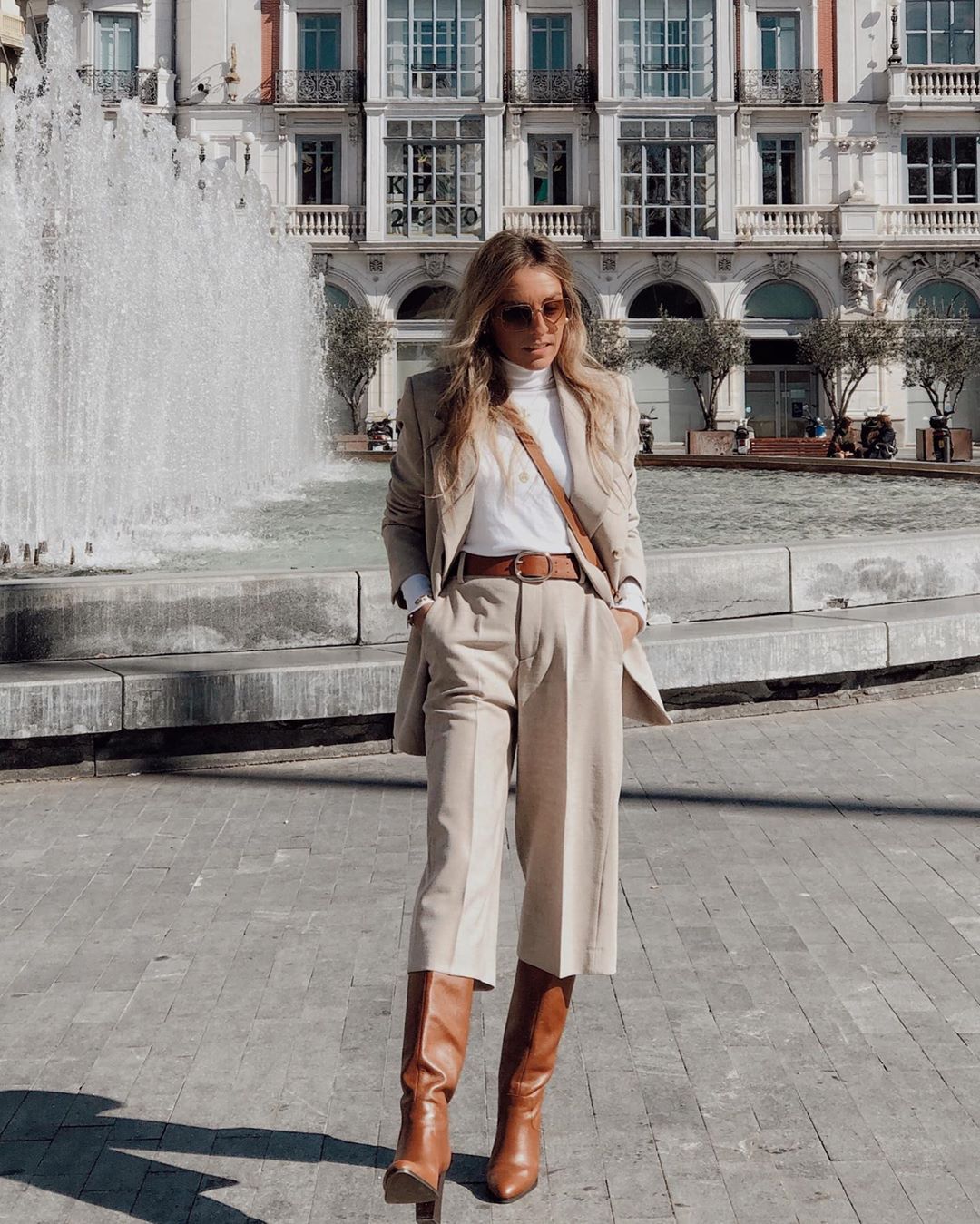In this daytime photograph, a fashionably dressed woman is captured mid-stride, her body angled slightly down and to the right as though walking toward the viewer. She is posed in front of an impressive mansion-like building painted white, featuring numerous glass windows. The mansion seems to boast multiple rooms and is likely quite sprawling. In front of this grand structure stands a large, circular fountain made of grey stone, slightly darker than the building. The clean, clear water of the fountain is seen rising well above the woman’s left side. Adding charm to the surroundings are trees positioned at the lower part of the image, along with benches encircling the fountain, all set on a brick-paved ground.

The woman’s attire is composed of a tan suit with a blazer and pants that fall just below her knees, complemented by a white turtleneck. Her accessories include a brown belt, brown boots, and a brown slingback bag with the strap crossing her chest, though the bag itself remains unseen. She wears tan sunglasses, and her hair—described as a shade somewhere between brown and dirty blonde—flows freely down to the middle of her chest. The primary colors featured in the photograph are various shades of brown and tan, combined with black, white, shades of grey, and blue. There's a noticeable absence of any text in the image.